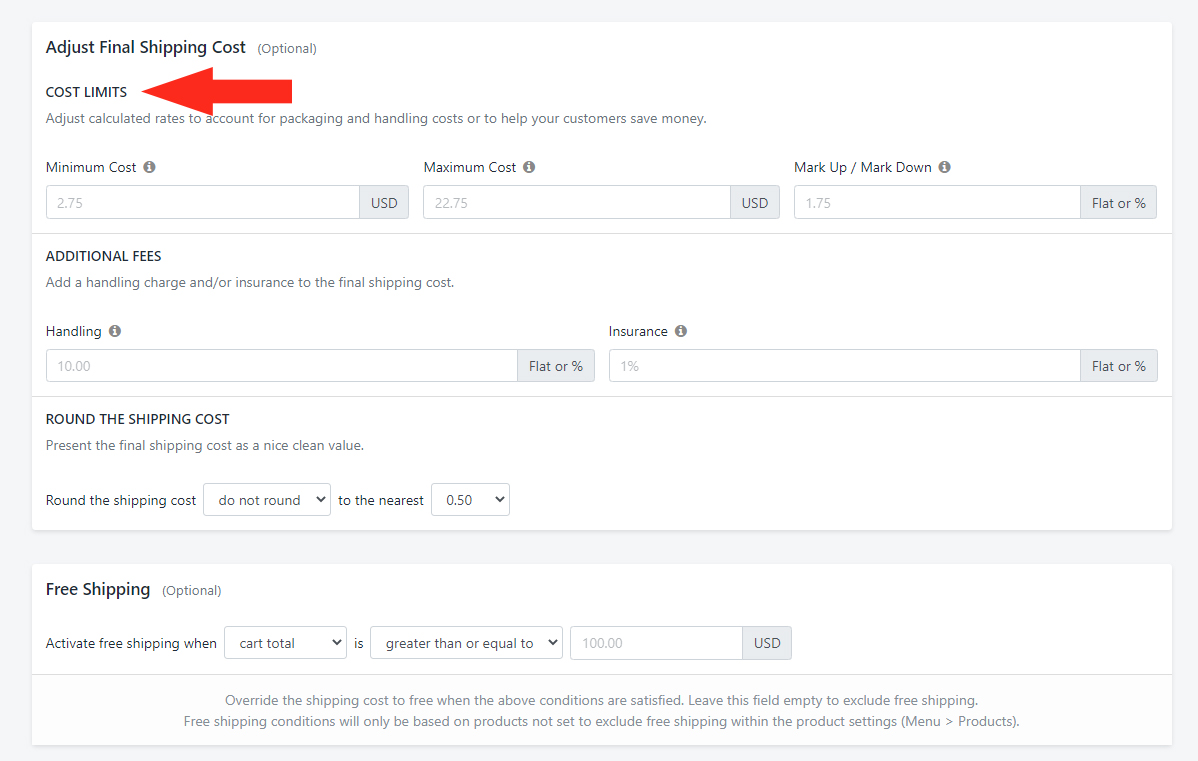**Caption:**

This webpage is a detailed shipping cost adjustment section on an e-commerce site, displayed in landscape orientation. The page features a pale gray border and a white background. In the top left corner, a prominent red left-pointing arrow with an arrow shaft directs attention to the "Cost Limits" section. Directly above, a heading in bold reads "Adjust Final Shipping Costs (Optional)."

Beneath, in smaller print, the text explains: "Adjust calculated rates to account for packaging and handling costs or to help your customers save money." Below this, various text entry boxes are available for inputting data. 

- "Minimum Cost" (U.S. dollars) with an info button next to it, currently defaulting to $2.75 in grayed-out text.
- "Maximum Cost" (U.S. dollars) defaulting to $22.75 in grayed-out text.
- "Markup/Markdown" field with an option to choose between flat or percent, defaulting to 175%, also in grayed-out text.

Further down, the "Additional Fees" section includes the ability to add handling charges and/or insurance to the final shipping cost. Two enterable text fields labeled "Handling" (defaulting to $10) and "Insurance" (defaulting to 1%) are each accompanied by a flat or percent selection option.

Next, there is a section for rounding the shipping cost to ensure a clean final value. A drop-down menu currently set to "Do Not Round" allows for altering this to round to the nearest chosen value, with 50 cents as the default option.

At the bottom, an optional section titled "Free Shipping" allows users to activate free shipping when the cart total is greater than or equal to a specified amount, which can be adjusted as desired.